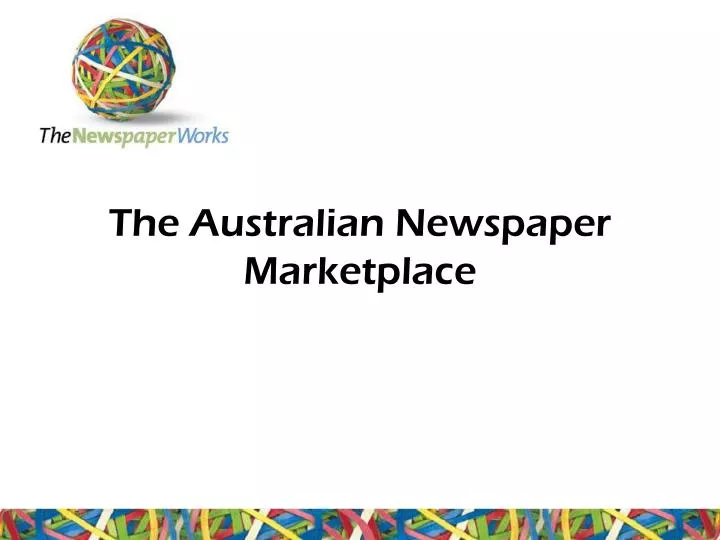The rectangular image serves as a slide or title page with a predominantly white background. A thin, horizontal banner of rubber bands stretches along the bottom edge, displaying rubber bands in colors such as yellow, white, green, lime green, pink, red, and light blue. Centered in the upper part of the image is black text in two lines: "The Australian Newspaper" on the top line and "Marketplace" on the second line. In the top left corner of the image, there is a rubber band ball, exhibiting a sphere formed by interwoven rubber bands in various colors, including yellow, white, pink, green, lime green, blue, light blue, and red. Positioned below this ball is a logo with the words "The" in black, "Newspaper" in green, and "Works" in blue.